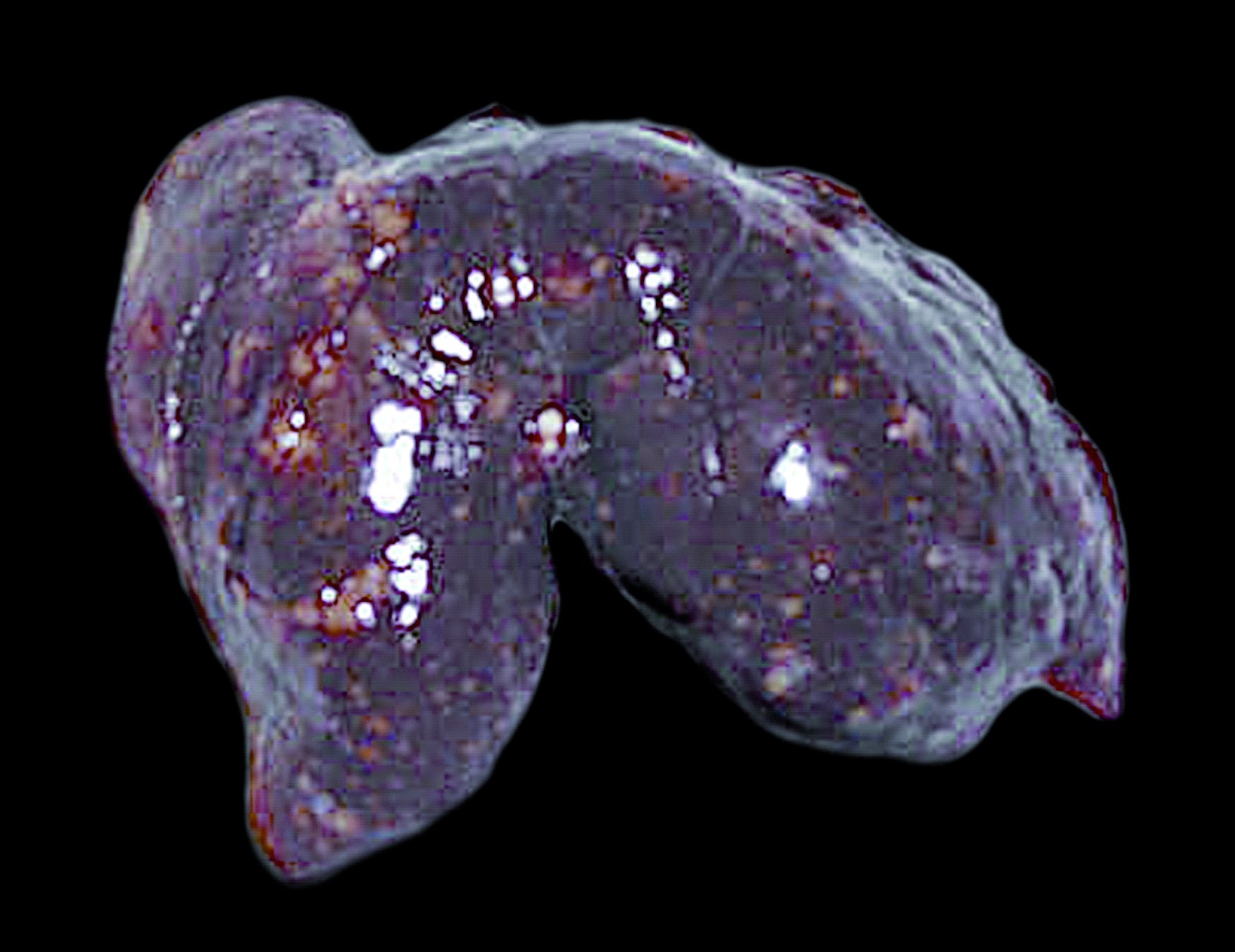In this striking image, a mysterious object takes center stage against a black background, making its intricate details and vivid colors stand out prominently. The object, predominantly a dark purple with grayish undertones, curves upwards in a shape reminiscent of a croissant or perhaps even a butterfly. It also has bright red accents and white details that suggest light reflecting off its surface, adding an ethereal quality. The object's texture and form could lead one to speculate it might be a uniquely shaped rock or even an exotic shell-like fish. Its vibrant hues of purple, lilac, and violet, combined with the interplay of light and shadow, create a visually captivating and beautiful composition.